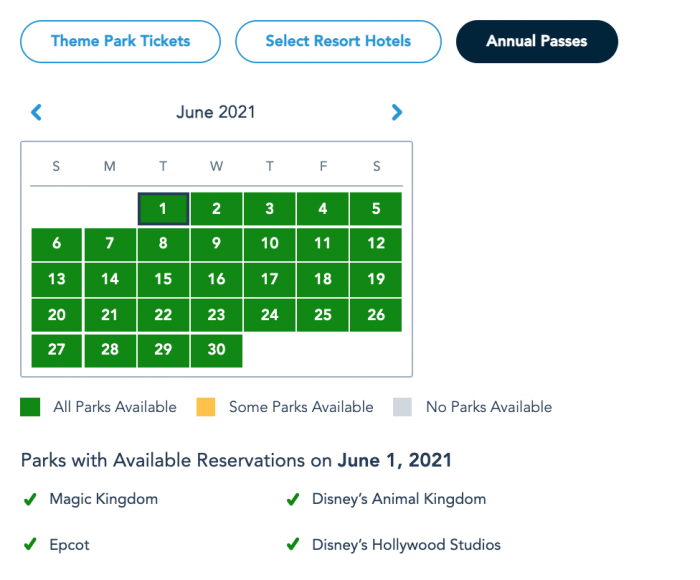This is a detailed screenshot of a webpage featuring a reservation calendar for June 2021. At the top, there are three pill-shaped buttons: two white ones labeled "Theme Park Tickets" and "Select Resort Hotels," and a black one labeled "Annual Passes." Just below these buttons, the calendar for June 2021 is displayed, accompanied by back and forward arrow buttons for easy navigation between months. 

The days of the week are represented by their initial letters, each enclosed in a green box with white characters. Below the days of the week, a legend explains the color coding: green squares indicate "All Parks Available," yellow squares signify "Some Parks Available," and gray squares denote "No Parks Available."

Under the legend, it lists the parks with available reservations for June 1, 2021. The parks available are: Magic Kingdom, Disney's Animal Kingdom, Epcot, and Disney's Hollywood Studios, each indicated with a green checkmark to the left.